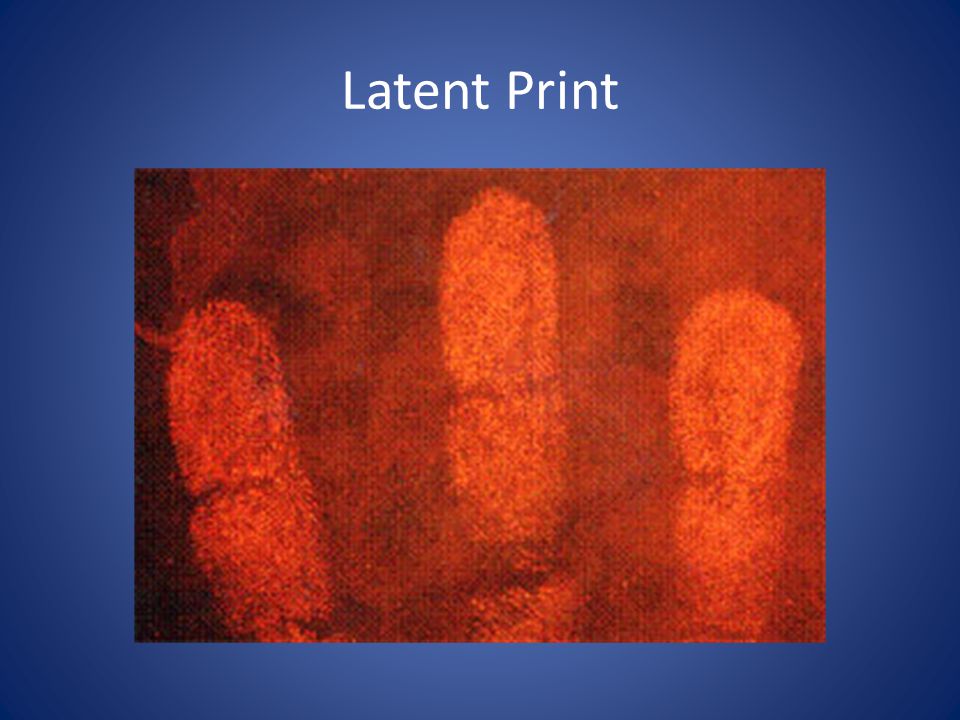The image appears to be a PowerPoint presentation slide with an almost abstract design. The background features a blue gradient, darker at the corners and lighter towards the center, giving a vignetted effect. At the top of the slide, in white font, the text "Latent Print" is prominently displayed, with each word capitalized. Below this text, there is a large, horizontally-aligned, orange rectangular image centered on the blue background. 

The central image depicts the top parts of three fingers - the index finger, middle finger, and ring finger - which appear to be making an impression on the orange surface. The fingerprints are rendered in brighter shades of orange, creating a visually striking contrast against the darker orange and brown tones of the background. The fingers are upright and evenly spaced, revealing details up to the second joints, similar to what one might see in an x-ray, but in warm hues. The overall effect is that of fingerprints illuminated under an orange light, corresponding with the “Latent Print” theme.